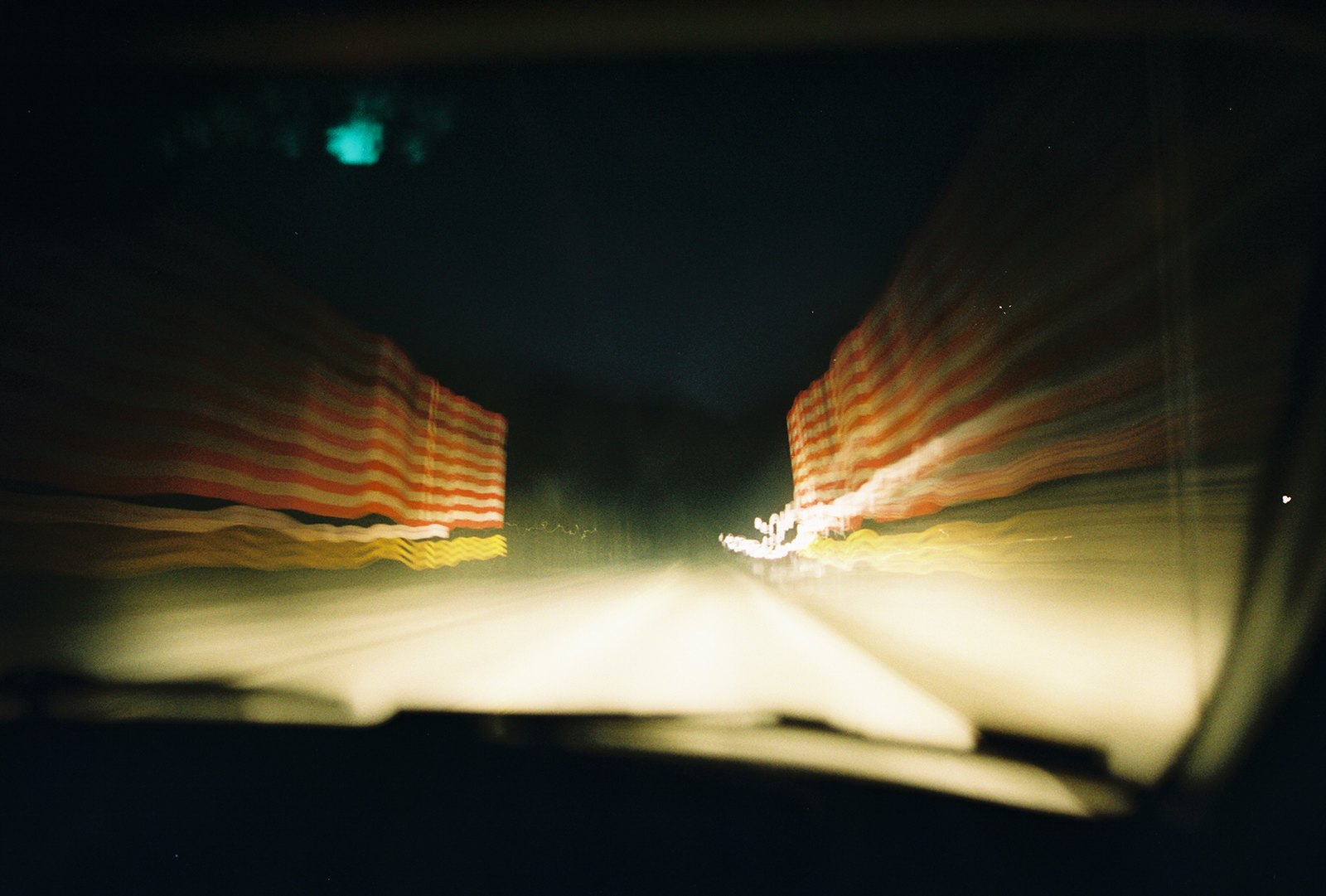This photograph, though blurry, depicts a car in motion at night, viewed from inside the vehicle, likely through the passenger side window. The road ahead is illuminated by the car’s headlights, casting a diffuse white light on its light gray surface. Flanking the road on both sides are structures with prominent white, red, and yellow striped patterns. The left structure visibly contains black elements at the bottom and transitions into white with red and yellow stripes. The right structure is similar but features a unique white strain running down its side. The sky overhead is predominantly black, punctuated by a cyan splotch on the left. In the distance, tall green weeds and leaves are faintly visible, adding an abstract touch to the night scene. The curved windshield features small black rectangle marks, further adding to the overall night-time ambiance.